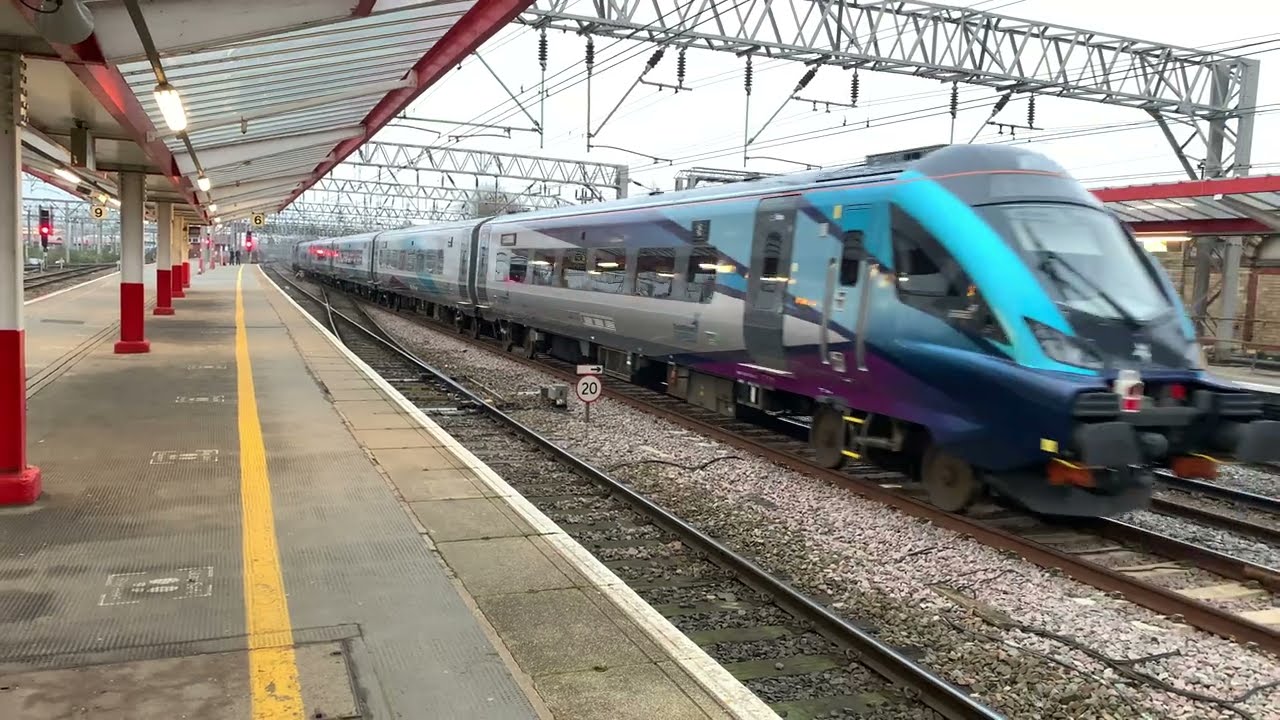In this detailed shot taken during an overcast day at an above-ground train station, a train is seen either parked or moving rightward through the frame, its front adorned in shades of blue and purple, and its body extending in silver hues. The platform from which the photo is captured features prominent red and white pillars supporting a metal overpass roof, with these pillars consistently lining the platform. The station's ground is distinguished by train tracks set in wood planks surrounded by rocks and pebbles, and a catwalk of metal frames can be spotted overhead. A circular sign with a red outline displaying "20" is visible to the left of the train. The platform is marked by a yellow line extending into the distance, beyond which glimpses of distant figures can be detected. The image captures the essence of an open, functional train station on a day enveloped by a gray, overcast sky, devoid of direct sunlight.